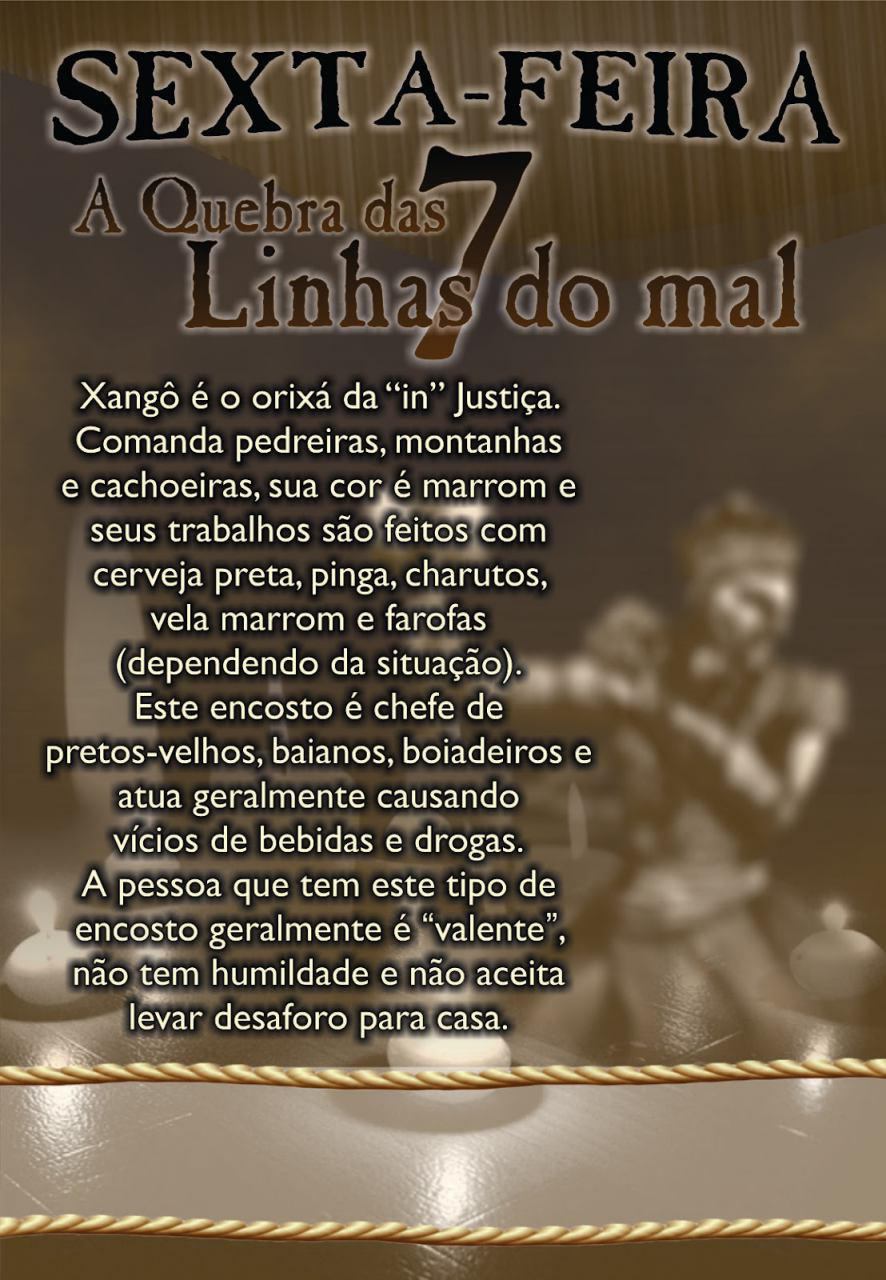The image features an intricately designed poster with a deep brown background. At the top, bold text reads "Sexta Feira" in thick, brown letters bordered in white. Behind the text are alternating dark and light brown vertical stripes that drape downwards, resembling a valence. Below this, another line of text spells out "Quebra Das Linhas do Mal," with a prominent number "7" integrated between the words. The font style of this text varies, with the number 7 being particularly eye-catching. The text below, which appears to be in Portuguese, starts with "Xango" and ends with "Casa."

The central background of the poster appears fuzzy, featuring a figure reminiscent of a soldier or an armored statue, potentially animated or 3D-rendered. Surrounding this figure are several lit candles. Along the bottom edge of the poster, two digital or drawn golden ropes extend horizontally, separated by a shiny gray area.